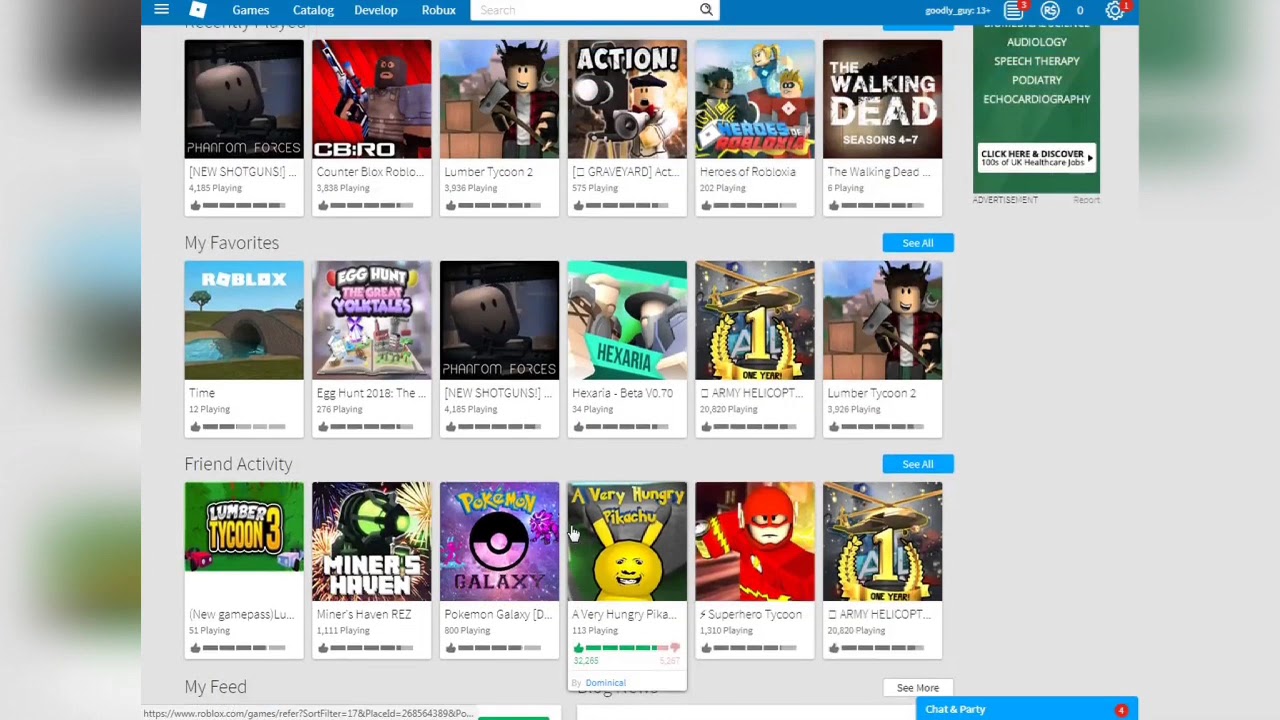This is a screenshot of a webpage from an online gaming platform, possibly Roblox. The interface showcases a variety of game options alongside their respective current player counts. At the top of the page, navigation tabs are labeled "Games," "Catalog," "Develop," and "Robux." The user is logged in as "Goodly_Guy," who is 13 years or older. 

Several game titles are prominently displayed with vibrant cover art. Featured games include:
- "Phantom Forces: New Shotguns," with 4,185 players currently engaged.
- "CB:RO (Counter Blocks: Roblox)," attracting 3,838 players.
- "Lumber Tycoon 2," hosting 3,936 players.
- "Action Graveyard," with 575 players.
- "Heroes of Robloxia," showing 202 participants.
- "The Walking Dead Seasons 4 through 7," with 6 active players.
- "Roblox Time," involving 12 players.
- "Egg Hunt: The Great Yolk Tales," popular with 276 players.

The screenshot also highlights various other titles such as:
- A duplicate of "Phantom Forces: New Shotguns," again with 4,185 players.
- "Hex Area: Beta V 0.70," engaging 54 players.
- "Army Helicopter," remarkably with 20,820 players.
- Another listing for "Lumber Tycoon 2," this time showing 3,926 players.

Additionally, a “Friend Activity” section lists:
- "Lumber Tycoon 3," showing 51 players.
- "Miner's Haven: REZ," with 1,111 players.
- "Pokemon Galaxy," hosting 800 players.
- "A Very Hungry Pikachu," with 113 players.
- "Superhero Tycoon," engaging 1,310 players.
- Another instance of "Army Helicopter," again with 20,820 players.

The bottom of the page includes options to "See More," "Chat," and "Party."